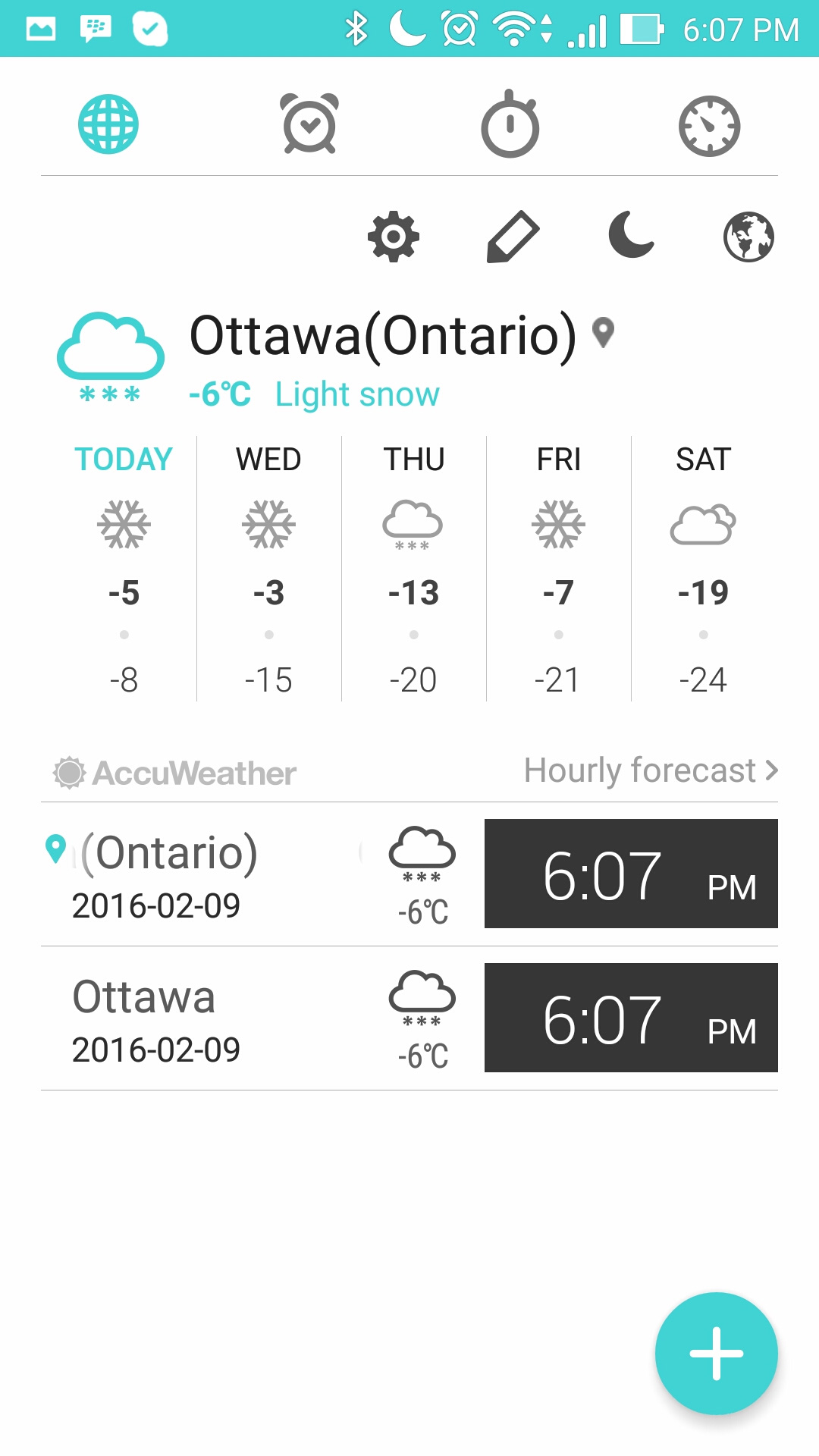The image displays a weather report on a cell phone screen, characterized by a blue border across the top. On the top left corner, there is an icon resembling mountains within a square with a white background. Adjacent to this, icons for Bluetooth, alarm clock, a moon indicating night mode, wireless signal, cellular connection, battery level, and the current time of 6:07 p.m. are visible.

Just below these icons, a series of additional icons are present: a globe, an alarm clock, a stopwatch, a regular clock, a gear, a pencil, another moon icon, and another globe icon. 

The main section of the screen shows a weather summary: a cloud icon with three snowflakes beneath it indicating light snow in Ottawa, Ontario, with a temperature of -6 degrees Celsius. Following this, a detailed forecast is provided for the upcoming days:

- Today: Snowflake icon, -5°C / -8°C
- Wednesday: Snowflake icon, -3°C / -15°C
- Thursday: Cloud with three snowflakes icon, -13°C / -20°C
- Friday: Snowflake icon, -7°C / -21°C
- Saturday: Cloud icon, -19°C / -24°C

At 6:07 p.m., as indicated in large print beneath the forecast, the weather information is summarized. The bottom of the page features a blue circle with a large white plus sign in the center, potentially for additional actions or settings.